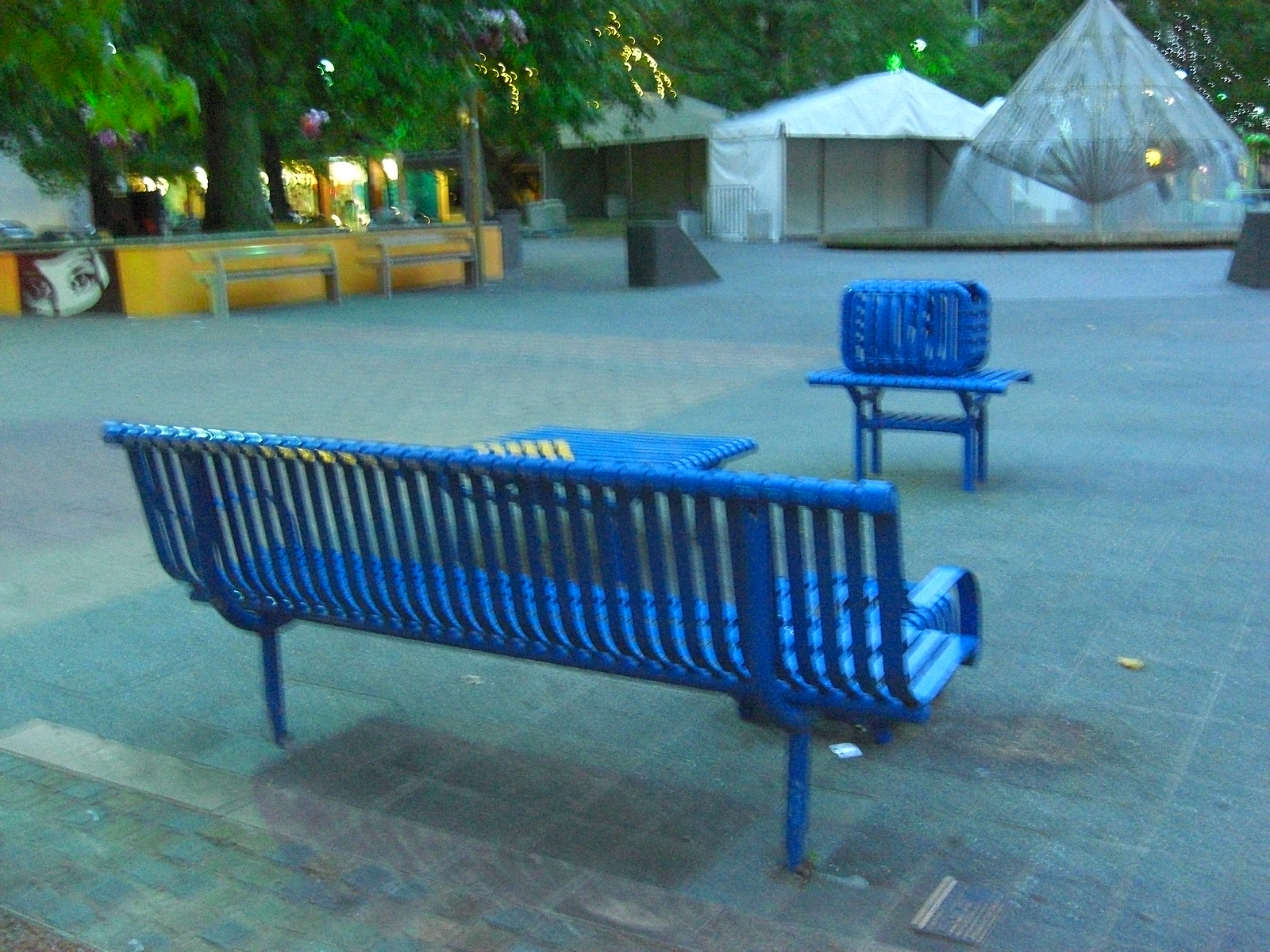This is a photograph of a somewhat blurry park courtyard set in an urban environment. The ground consists of a large square of cement with accents of brown-colored blocks. In the bottom left corner, there is a long metal cornflower blue bench with railings on the back, through which we can see. Directly in front of the bench sits a matching blue metal table, and beside it, a small low table of the same color holding a large blue cube. In the upper left quadrant of the image, a yellowish stone wall stands with two benches placed against it, and a large tree rises behind the wall. The tree canopy is adorned with fairy lights, giving the impression that it may be evening. In the far upper right, several canvas-style pop-up tents suggest that a fair or event might be taking place. The tents are framed with a backdrop of green shady trees. Additionally, on the pavement in the upper right section, there appears to be an unusual, possibly diamond-shaped object, which might be a fountain, covered with a layer of plastic.